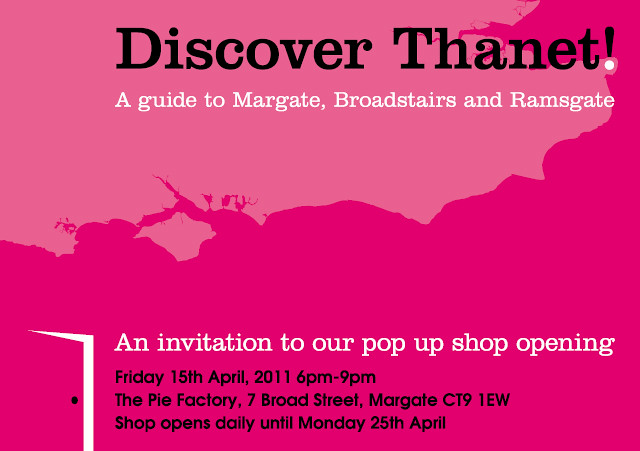This image appears to be an invitation for an event, set against a landscape-oriented background fading from light pink to dark pink with a shadowy, tree-like design. At the top, bold black text reads "Discover Thanet," followed by "A Guide to Margate, Broadstairs, and Ramsgate" in white letters. The central portion of the image is a seamless blend of light and dark pinks with no additional imagery. Towards the bottom, an invitation in white text announces, "An Invitation to Our Pop-Up Shop Opening," followed by the details in black text: "Friday, 15th April, 2011, 6 p.m. to 9 p.m., The Pie Factory, 7 Broad Street, Margate, CT9 1EW." The shop is noted to be open daily until Monday, 25th April. There are no specific indications of what type of shop it is, though the name "The Pie Factory" might suggest a focus on pies or baked goods. The overall design is minimalistic, with an intriguing detail in the bottom left corner resembling an open doorway with a black doorknob, adding to the invitation's allure.